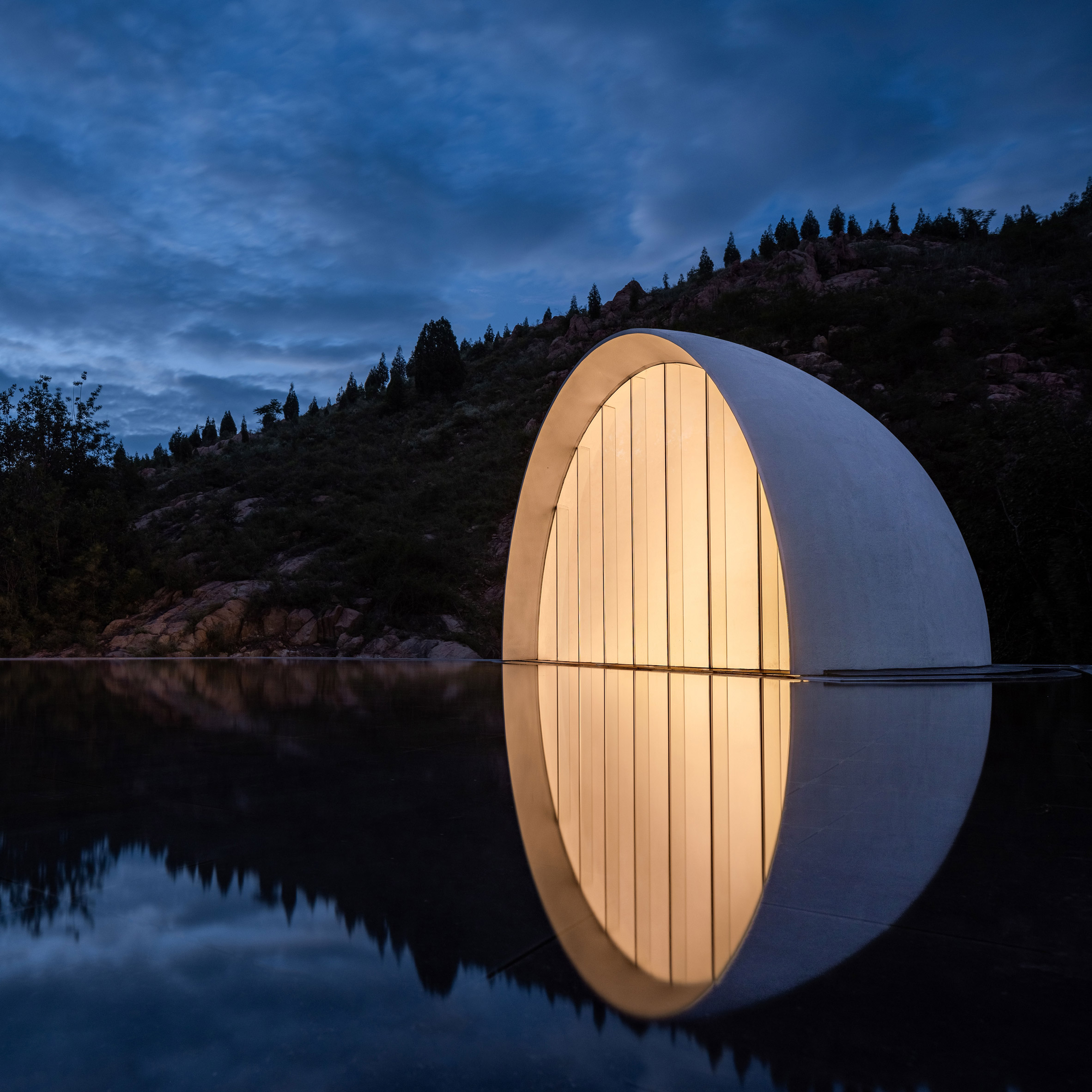The image captures a mesmerizing, modern scene at dusk, showcasing a large, illuminated semi-circular dome on the edge of a perfectly still body of water, most likely a lake. The dome's lighted exterior shines with a soft, warm yellow hue, enhanced by vertical lines which may be opaque panels, adding a distinct architectural character. This lighting creates an exact mirror image on the water, forming an illusion of a complete glowing circle. The sky above is tinged with a dark blue, scattered with greyish clouds, indicating twilight. Behind the dome, a hill dotted with trees and boulders rises, with its slopes partly obscured by the fading light. The shore at the water’s edge is lined with what appears to be brownish rocks, contributing to the rugged and serene landscape. The scene evokes a luxurious, tranquil atmosphere, typical of high-end glamping experiences.